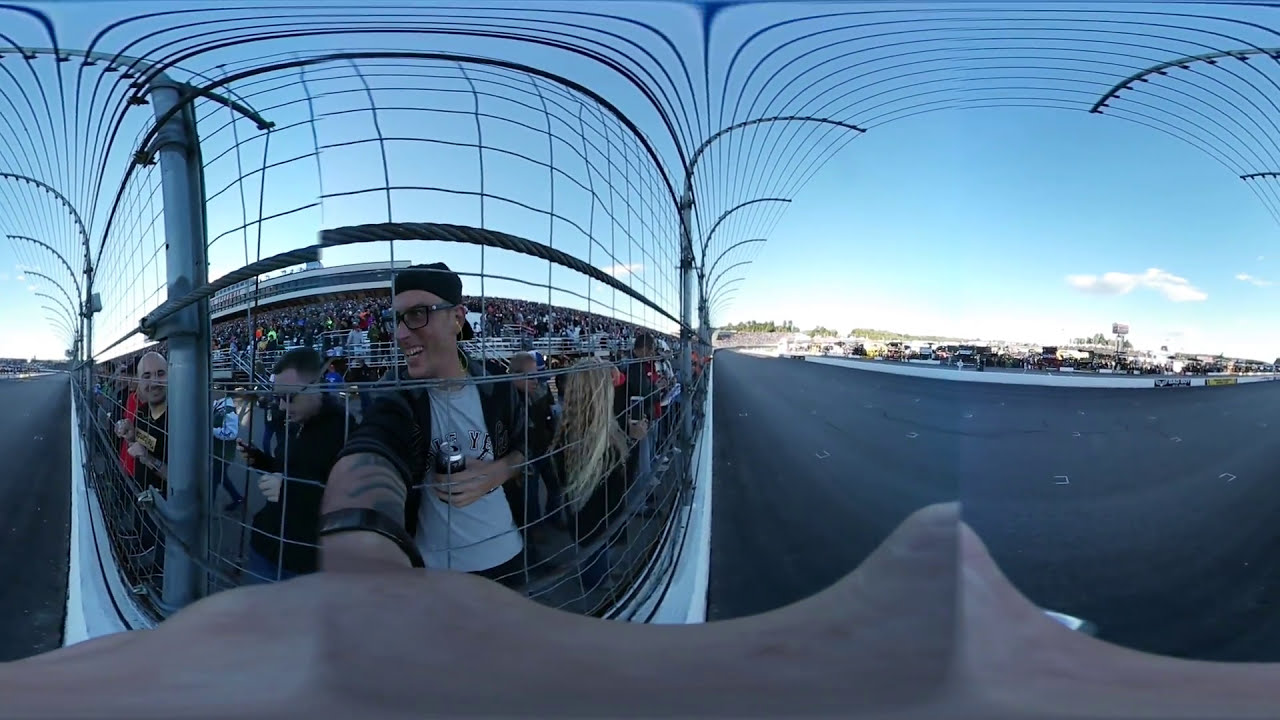The photograph is a panoramic fisheye selfie taken by a man at what appears to be a NASCAR or car racing track. On the left side of the distorted image, the man in question is visible, sticking his right hand through a chicken wire protective fence to hold the camera. He is wearing a black baseball cap facing backwards, black framed glasses, a short-sleeved button-up shirt left unbuttoned with a gray shirt underneath, and a black wristband on his right wrist. In his left hand, he holds a beer can. The racetrack, a solid black tarmac surface, is separated from the audience by a small white wall, the chicken wire fence with a slightly curved top, and tiered seating with multiple spectators. The photograph captures a sunny but late day, as the area on the right is bright while the left side, including the track and audience, is shaded. No race cars are visible on the track.